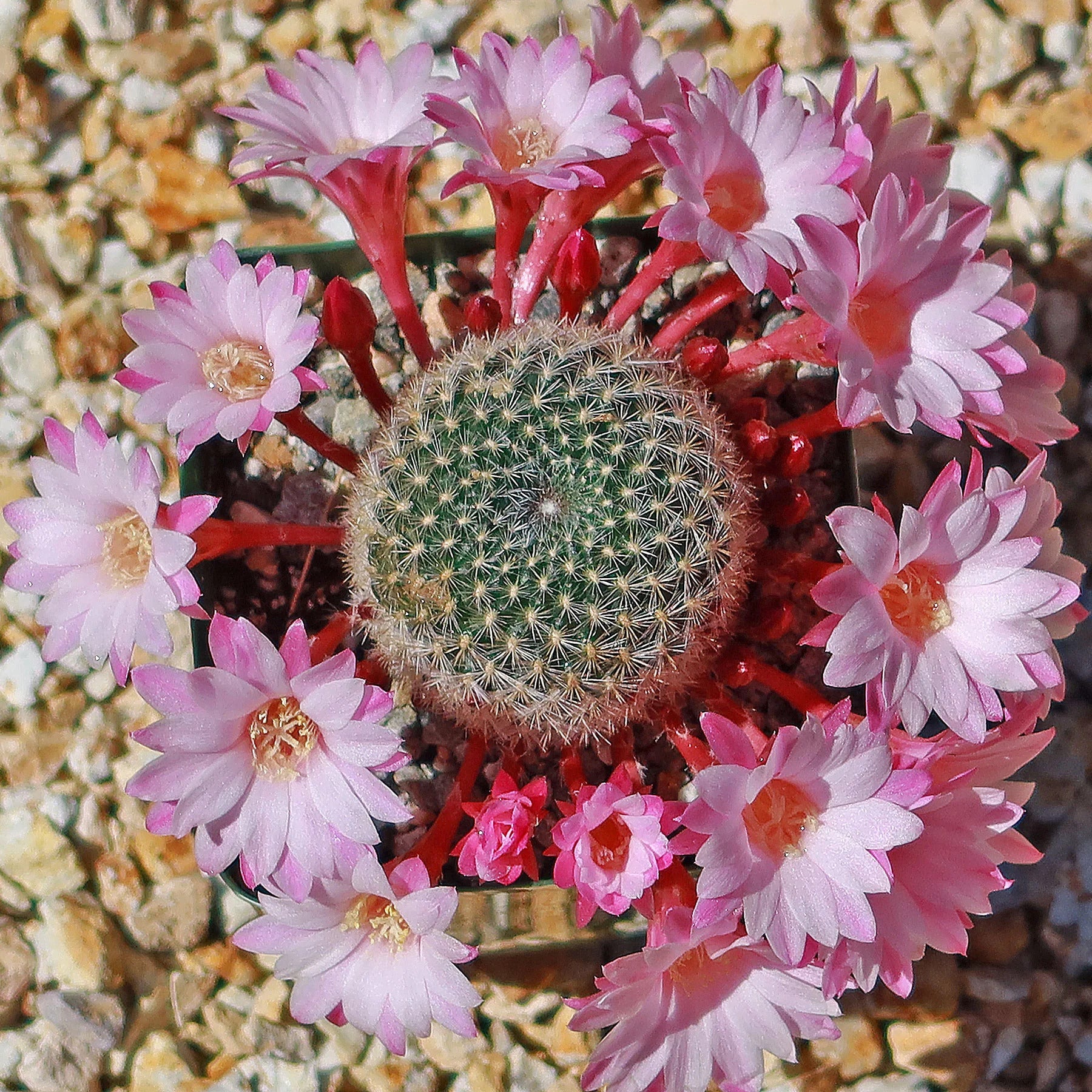The image presents a top-down view of a round, ball-shaped cactus with fine white thorns, each sporting a delicate circular twist towards the center where a little white dot resides. Encircling the cactus are numerous blossoms featuring maroon-colored stems that emanate from beneath the cactus, extending outward. The flowers themselves boast layers of light pink petals tinged with hints of purple, with numerous white pistils and stamens protruding from their centers. The entire composition is situated within a green, square pot, which rests on a bed of small, clean gravel stones in shades of tan and brown, providing a modern yet natural backdrop for the vibrant cactus and its delicate flowers.